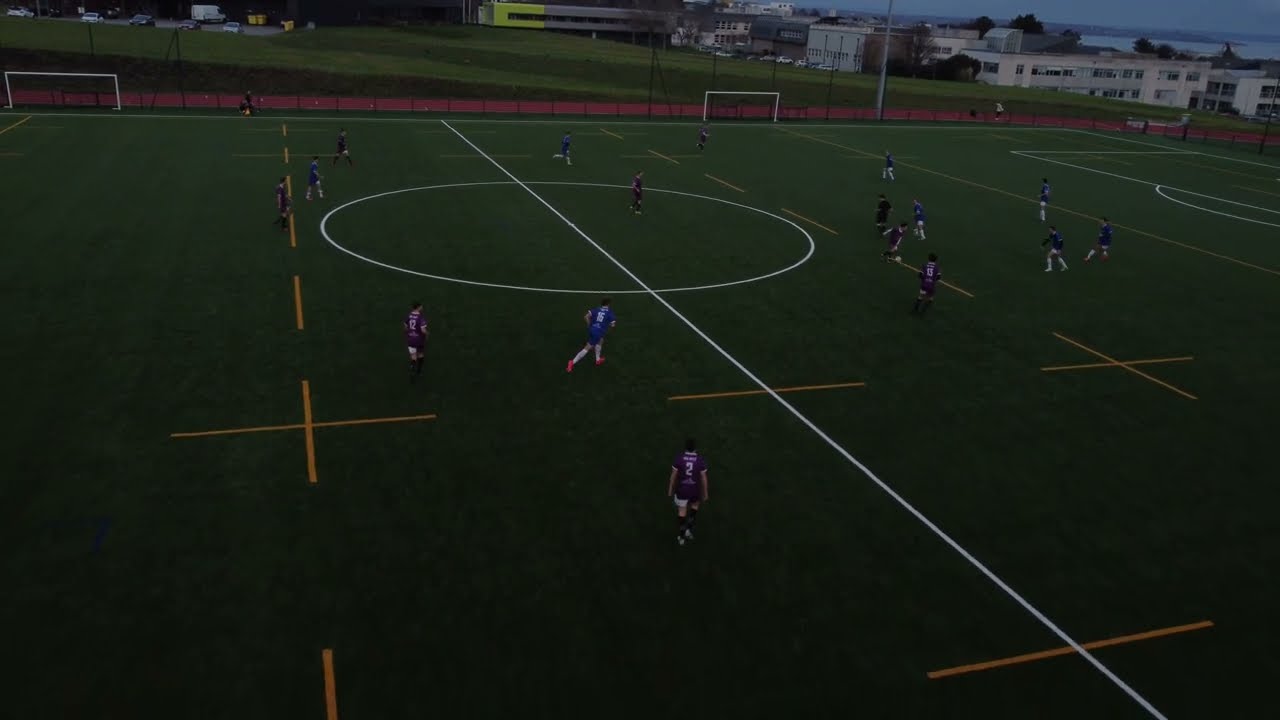The image depicts an outdoor, open-air soccer field taken at dusk, creating a dimly lit scene suggestive of late evening or approaching stormy weather. Central to the image are numerous soccer players actively engaging in a game. The players are divided into two teams: one team donning all-blue uniforms and the other wearing purple uniforms. A referee dressed in black is also visible. The field itself is marked with white and yellow lines, including a diagonal line and a central circle. Encircling the field is a red running track. Beyond the track, the scenery expands to a green grassy area, with buildings visible in the top right corner of the image. Additionally, a body of water and a sliver of the sky are also discernible in the backdrop. The image is rich with colors, including green, yellow, purple, blue, white, black, lime green, and tan, providing a vivid yet serene depiction of a sports field in action.